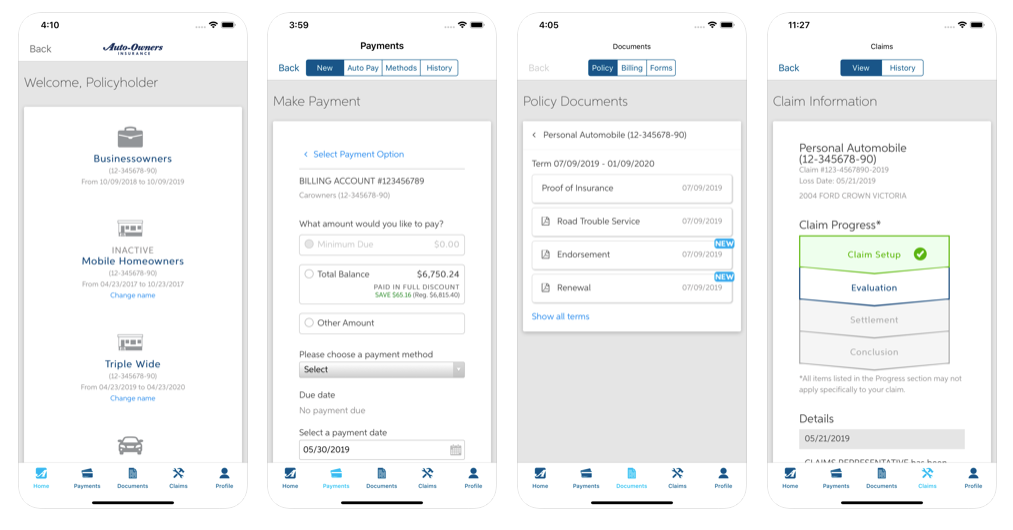This image is a compilation of four sequential screenshots, each depicting different sections of a mobile insurance application interface. 

The first screenshot features the main dashboard of the Auto-Owners Insurance app. At the top, the header reads "Auto-Owners Insurance" with a timestamp of 4:10, a full battery icon, and an active Wi-Fi symbol in the upper left corner. The center of the screen prominently displays "Auto-Owners Insurance" in bold text. Below it, a light gray banner welcomes the policyholder. The middle section of the screen shows two notable options in blue text: "Business Owners" accompanied by a briefcase icon and "Mobile Homeowners" paired with a house icon.

The second screenshot showcases a menu interface with four tabs: "New," "Auto Pay," "Methods," and "History." The "New" tab is highlighted. Below the menu, there is an option to "Make Payment" in a white box, and beneath that, a link to "Select Payment Option" highlighted in blue. The screen then asks, "What amount would you like to pay?" with an input box for entering the amount. It also displays a total balance due of $6,750.24. At the bottom, there's a prompt to "Please choose a payment method" with a dropdown menu for selection.